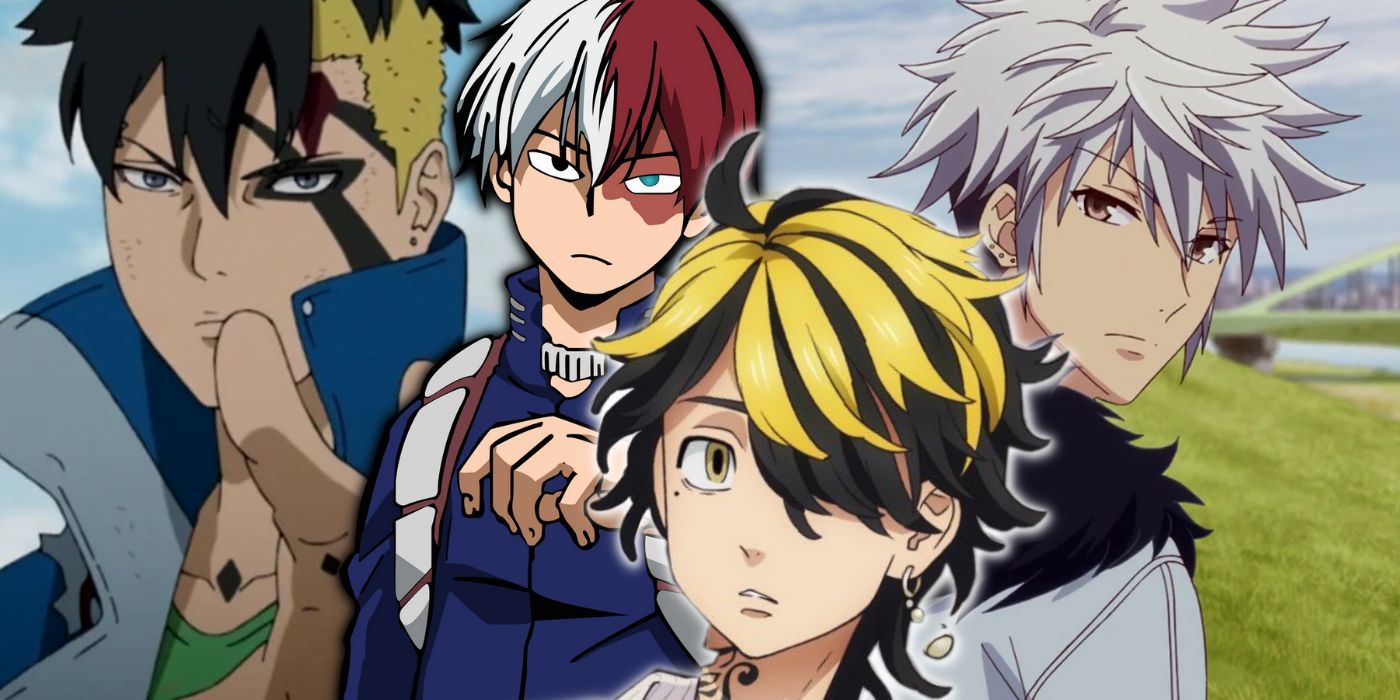The rectangular image, in comic book style, depicts four anime characters set against an outdoor backdrop featuring grass and a blue sky. The characters appear to be of Asian descent and have serious, intense expressions.

1. The character on the left has long black hair sweeping down across the forehead and two distinct black scars on the left side of his face.
2. Next to him is a boy with striking hair divided into white on the left side and brownish-red on the right, dressed in a blue jacket.
3. The third character, positioned more in the foreground, is a girl with a surprised or sorrowful expression, sporting black and gold (blonde) hair and wearing a brown earring. Her standout feature is her hair that has black sections interwoven with blonde highlights.
4. The final character, located to the right, is a boy with light grey, fluffy hair, dressed in a light blue jacket.

All characters are gazing directly at the viewer with serious, somewhat menacing expressions, creating a dramatic atmosphere for the scene.